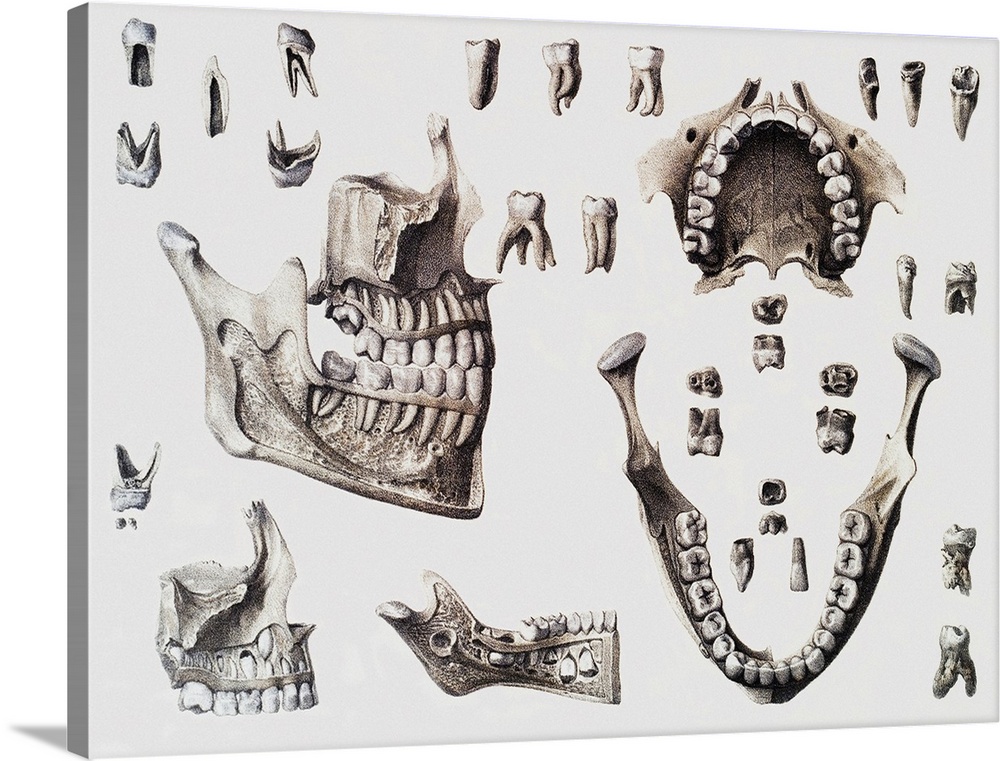The image is a detailed, computer-generated artistic representation of dental anatomy, resembling a medical diagram that a dentist or dental enthusiast might appreciate. This black and white print features an assortment of teeth illustrations meticulously articulated in various ways. 

On the left side of the image, there is a comprehensive depiction of an entire mouth, showcasing both upper and lower sets of teeth. On the right side, the upper half of the teeth is presented above, while the lower half is illustrated below. Surrounding these main sections are individual drawings of teeth and cross sections that include intricate details of tooth roots, gums, and bone structure. 

The diagram also includes representations of child teeth, showing how adult teeth grow in from underneath. The various cross sections—from top down, bottom up, and from the side—capture the complexity of the jaw and teeth development. This captivating piece of art is organized on a standout poster board, presenting a thorough exploration of dental anatomy.